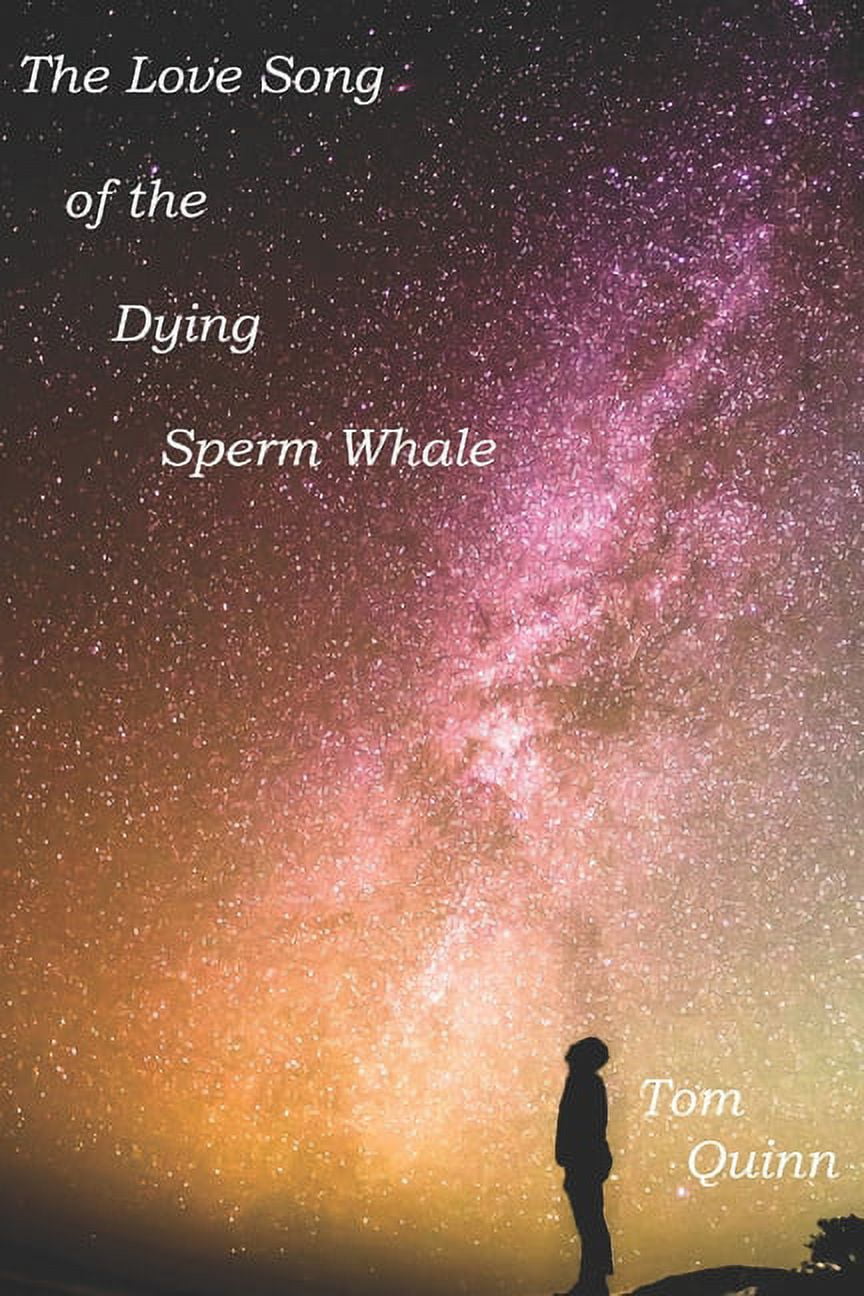The image is a richly detailed poster or book cover titled "The Love Song of the Dying Sperm Whale" by Tom Quinn. The title, written in elegant white font, is positioned in the upper left corner against a dramatic night sky. This sky transitions from a deep black-blue in the top left to mesmerizing shades of beet red, magenta, burnt orange, and pale yellow as it descends and moves right, giving the impression of a celestial event or a nebula. 

In the center, a large galaxy, possibly the Milky Way, arcs gracefully with a prominent purple nebula bleeding into golden and pink hues. Hundreds of tiny stars are scattered across this colorful backdrop, evoking a sense of endless space and mystery.

At the bottom right, standing on a small hill, is the silhouette of a man looking up in awe at the sky. Nearby, the faint outlines of a tree and possibly a small house add depth to the scene. The author's name, Tom Quinn, is written in white text next to the man's silhouette, tying the serene yet captivating imagery together. 

This composition creates a visual narrative that invites viewers to gaze into the cosmos and contemplate the story hinted at by the evocative title.